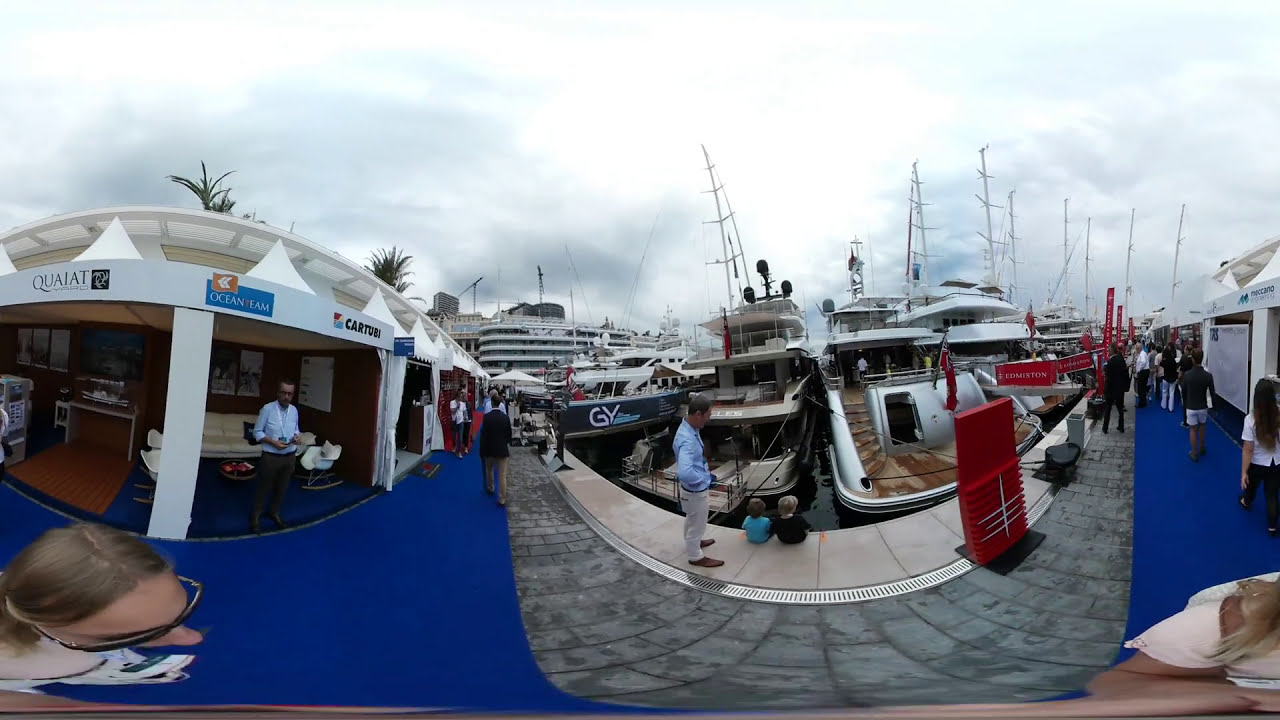Captured through a fisheye lens that bends the straight lines of reality, this panoramic image of a bustling boatyard reveals a dynamic scene filled with details. The scene centers around numerous boats clustered together, their masts piercing the cloud-filled sky. A large multi-story ship equipped with cranes sits towards the left background, towering over the smaller vessels. The walkway, constructed of gray planks, forms a U-shape, bordered by a blue path where a few people stroll, creating a lively atmosphere.

On the left and right sides of the image, the lens's distortion causes warping, adding an unusual dimension to the view. The left side of the walkway features a standout figure— a person with light brown hair, parted in the center, wearing sunglasses. Nearby, a man in a white shirt and black pants stands in the entrance of a building, with a white couch visible behind him.

Further detailing the human activity, a woman with long black hair in a white shirt walks methodically, while close by, a person in a black shirt and white shorts strides towards the right side of the walkway. Amid the vibrant scene, two children sit on the edge of the pathway, engrossed in watching the boats, with an adult guardian nearby.

Notably, signage above covered seating areas spells out "QUAIAT," "OCEANFAM," and "CARTUBY," suggesting potential store names or attractions. Numerous people move about, possibly participating in a boat show or simply enjoying a day by the waterfront.

The overall image carries a distinct virtual reality or 360-degree feel, emphasizing the surreal bent lines and overlapping spaces. The sky above completes the tableau with a mix of heavy, lumpy clouds interspersed with patches of light blue, encapsulating the vibrant, bustling essence of the boatyard.